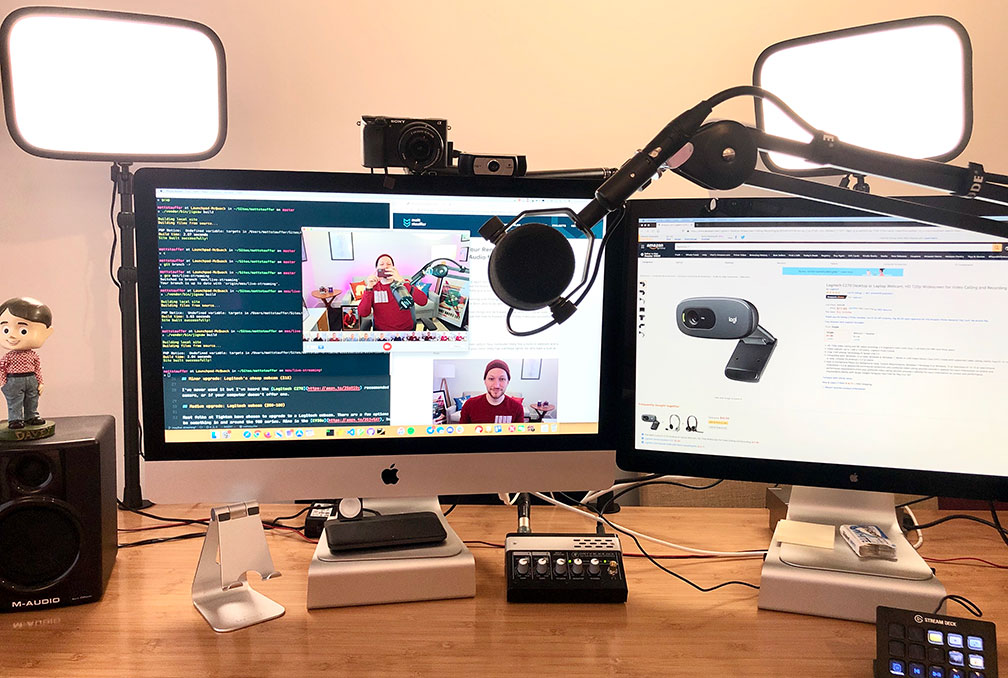The image depicts a detailed office desk setup featuring advanced computer equipment. Centrally, there are two large monitors both powered on and displaying different contents. The left monitor shows a Zoom call with two participants, their faces occupying small squares on the screen amidst unreadable text on a dark background. The right monitor displays a webpage filled with text, likely describing a device featured on the white backdrop. Above the monitors, two bright square lights illuminate the setup, aiding in clear video capture.

On the wooden desk, light in color and grain, sits a range of devices and accessories. To the left of the monitors, a small brown speaker supports a whimsical bobblehead figurine dressed in a checkered shirt and jeans. Nearby, a substantial microphone stands prominently in the middle of the setup, indicating frequent audio or video conferencing. Adjacent to this are various control panels and pieces of recording equipment, suggesting a comprehensive and well-used multimedia workspace. A large webcam affixed to the top of the left monitor completes the arrangement, signifying a space designed for both communication and content creation.